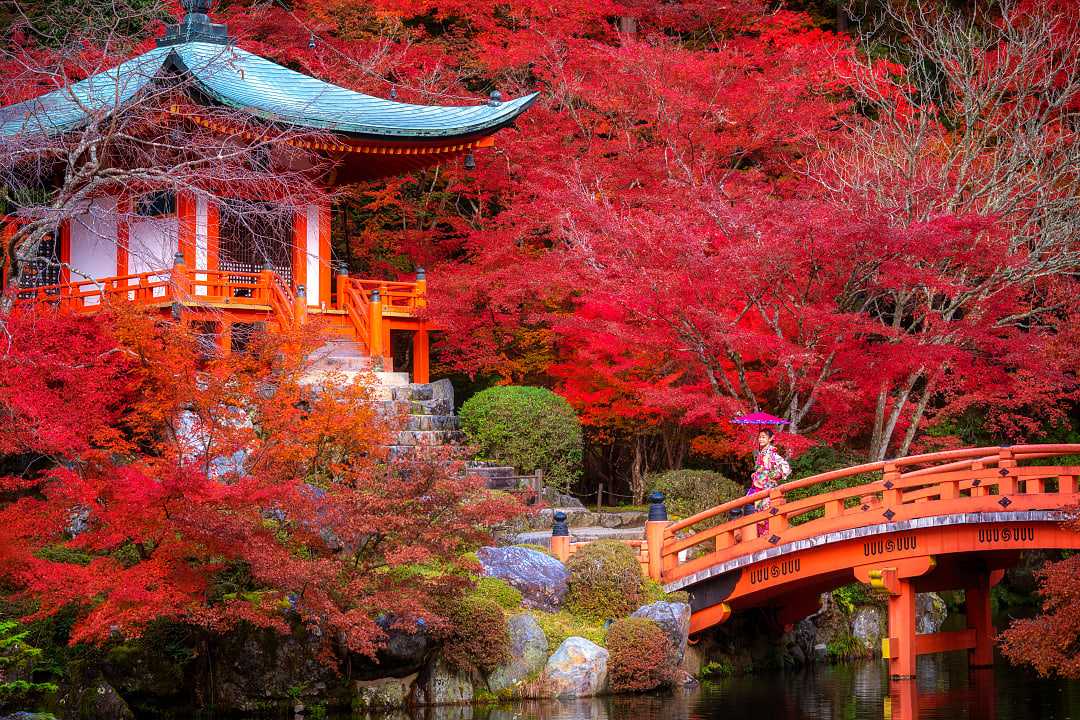This image captures the serene beauty of a traditional Japanese temple set within a lush garden. Dominating the scene is a picturesque orange bridge, arching gracefully over a tranquil body of water. Two women, dressed in exquisite floral gowns and carrying ornate umbrellas—one pink and the other purplish—are crossing the bridge, adding a touch of human presence to the peaceful setting. The temple itself, nestled in the upper left of the composition, features a distinctive blue-tiled roof with gentle curves, and an orange and white structure that likely houses a shrine. Leading up to the temple are several staircases, inviting visitors to ascend. The foreground is adorned with green bushes and scattered rocks, while the background bursts with vibrant colors from trees with red and orange leaves. Some of the trees are bare, adding a seasonal contrast to the lush foliage. The overall ambiance of the photograph is tranquil and calm, vividly capturing the essence of a traditional Japanese garden.